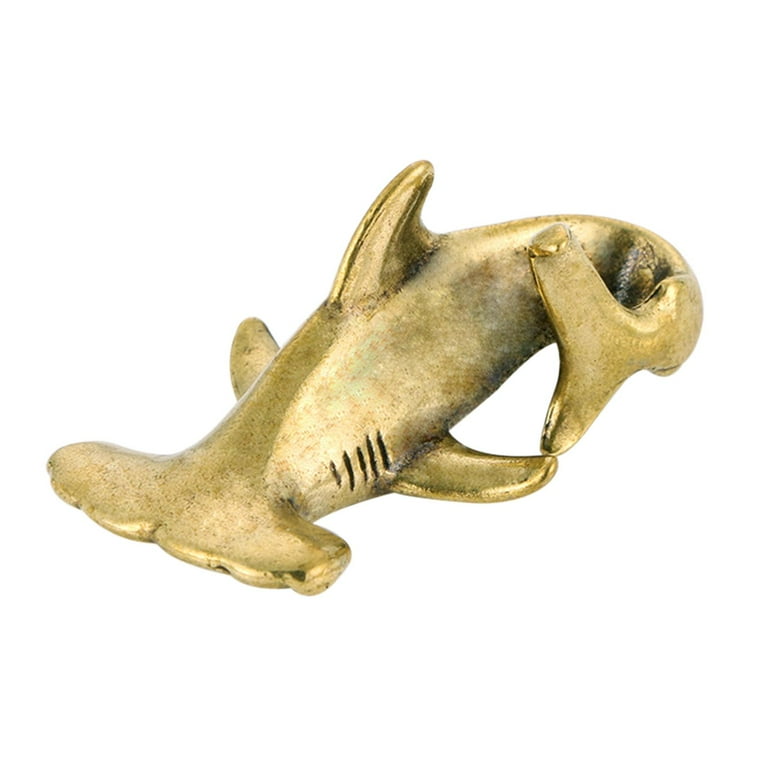This image features a detailed gold and bronze-colored hammerhead shark sculpture set against a white background. The sculpture has a somewhat cartoonish appearance, with notable hammerhead features and an oblong-shaped head adorned with small indentations. The body showcases side and dorsal fins, and the tail is gracefully curved to touch one of its side fins. The shark's body bears speckled patterns of black and white, particularly noticeable on its underside. Dark slits indicative of gills are visible on the left side, providing additional detail. The sculpture, resembling a collectible or mini figurine, emanates an impression of weight and craftsmanship, highlighted by a mix of gold, orange, and rust hues, giving it a goldish-green tint.